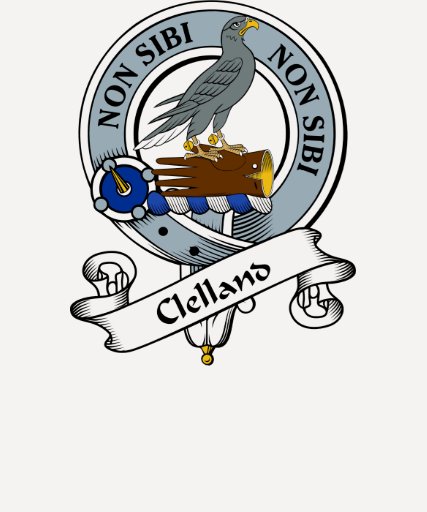This image depicts a detailed crest for an organization, featuring an emblematic bird and structured text. At the center is a gray bird, likely an eagle, adorned with two bells on its legs and perched atop a brown falconry glove. The bird has a yellow beak and is gazing upward, head tilted back. This entire scene is framed by a gray ribbon inscribed with the Latin phrase "Non sibi, non sibi" twice, forming a circular ring around the bird.

The glove rests upon an alternating blue and white rope that extends toward a blue shield. The shield is outlined in white and features gray dots in each of its four corners, with a yellow spike or compass needle pointing due northwest from the shield’s center. Below this complex assembly, a white sash is prominently displayed with the text "CLELAND" in black letters, suggesting the crest may represent a family name or an organization's emblem. The intricate design elements and the specific symbols suggest a rich tradition or long-standing heritage, potentially linked to a specific group or society.